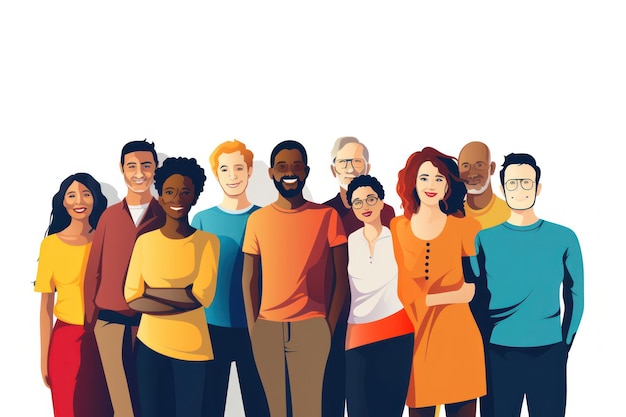In this animated image of a diverse group of ten smiling individuals, we see a mix of men and women spanning various ages and races, dressed in vibrant and polychromatic clothing. At the front, a Hispanic-looking woman stands out in a yellow blouse and red dress. Beside her is a European man with black hair, dressed in a brown tunic shirt over a white t-shirt and tan pants, and a black woman with her arms folded, wearing a white blouse and black pants. A young red-headed white man smiles in a blue t-shirt and black pants, and next to him, a slightly older black man with black hair and beard beams in an orange shirt and brown pants. Another Hispanic-looking woman with eyeglasses and curly black hair wears a white blouse with an orange stripe and black pants, while a white woman with red hair and bright red lipstick dons an orange dress with black buttons. Standing behind them are two older gentlemen: a white man with glasses, gray hair, and a beard, dressed in a teal shirt and dark pants, and a bald black man with a white or gray beard. Everyone in the group exudes happiness and camaraderie, reflecting a community enriched by its diversity and colorful attire.